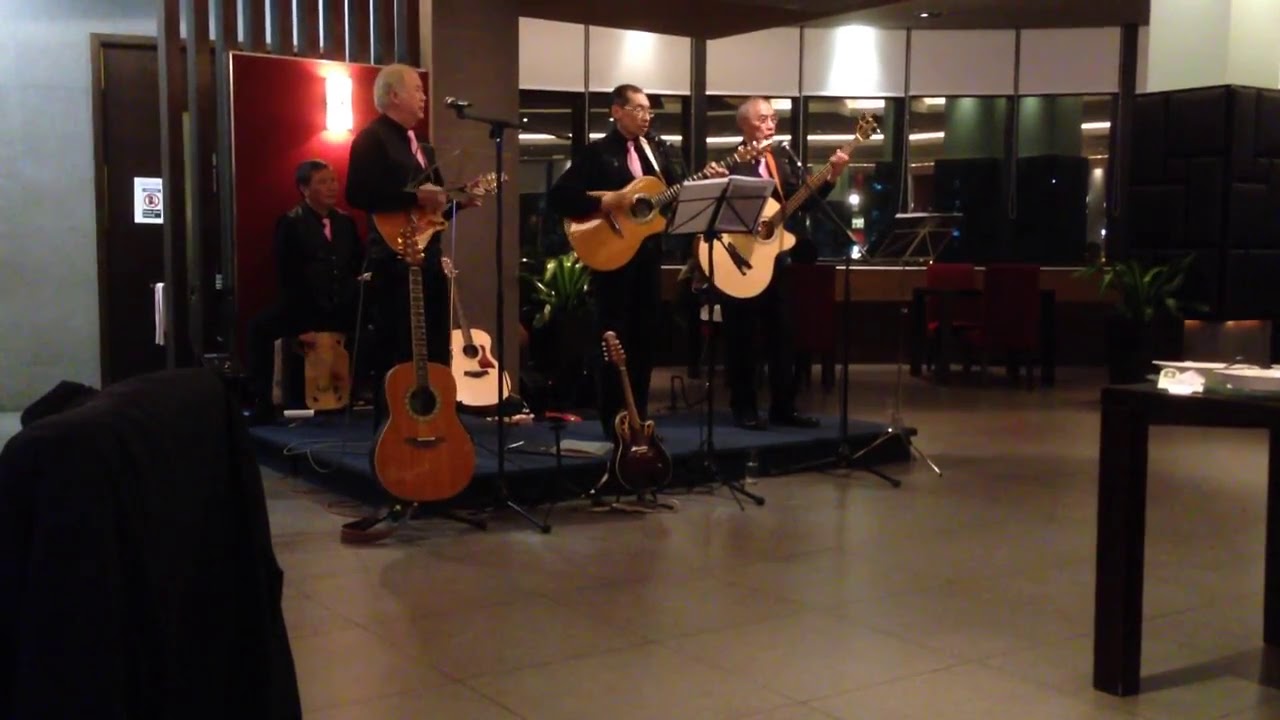In this indoor scene, a band consisting of four older gentlemen, possibly in their 60s or 70s, are performing on a slightly elevated, portable blue stage. The band members, who appear to be of Asian descent, are all dressed uniformly in black suits with pink ties and matching black pants. At the front of the stage, three men stand close together, each with his own stringed instrument: the man on the far right holds a light tan acoustic guitar, the man next to him holds a light brown acoustic guitar, and the third man holds a small ukulele. All three have microphones placed in front of them for singing.

Behind these three musicians, a fourth man sits on a stool, partially obscured by the performers in front of him. He is also dressed in a black suit with a pink tie. It is unclear whether he is playing an instrument, possibly drums, as he is mostly hidden from view. 

The setting includes some additional elements like guitars placed in front of the stage, a music stand, windows with lights to the right, and what appears to be a bag for their equipment to the left. The room's floor is covered in light tan tiles, and there are some tables with speakers or recording equipment scattered around. The rear of the stage features a red screen, adding a contrasting background to the performance area.